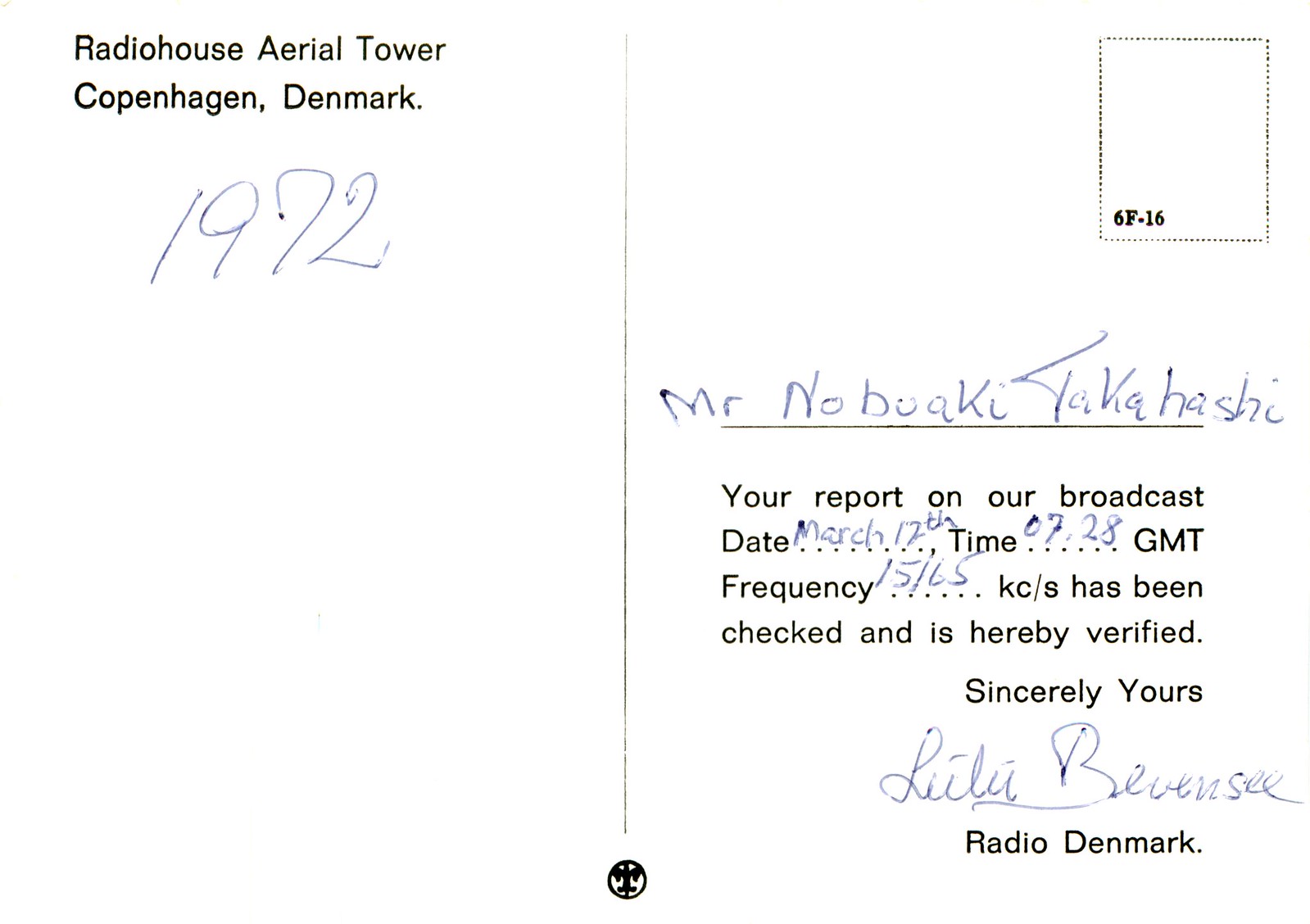The image features a vintage black-and-white postcard, titled "Radio House Aerial Tower, Copenhagen, Denmark, 1972," written in black text on the upper left. Handwritten in blue ink, 'Mr. Nobaki Takahashi' is noted towards the right, where a blank postage area is present. Below the inked name, a formal note printed in black text reads: "Your report on our broadcast date March 12th, time 0728, GMT frequency 15165 KC/S has been checked and is hereby verified." It is signed, "Sincerely yours, Lily Bevensie." The postcard ends with the text "Radio Denmark" and features a small logo beneath a number on the left.